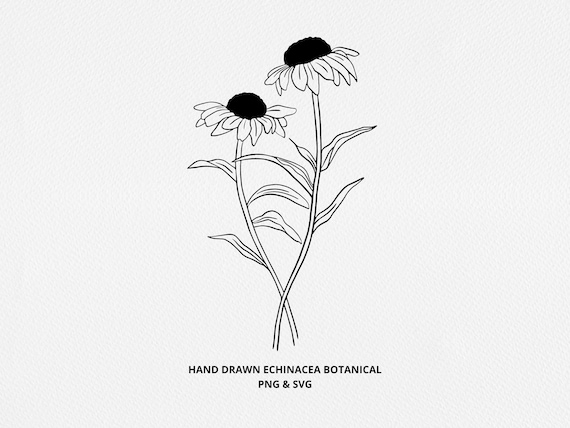This black and white illustration features a hand-drawn botanical sketch labeled "Hand-drawn Echinacea Botanical" with additional labels PNG and SVG beneath it. Dominating the center of the image are two slightly intertwined, overlapping flower stems, each adorned with multiple leaves. The stems begin crisscrossed at the bottom and stretch upward, nearly reaching the top of the picture. The flowers bear resemblance to both daffodils and daisies, each with distinct petals and a central bud. The left flower stem has three leaves, while the right one appears slightly taller with a varying number of leaves. The entire illustration is set against a stark white background, emphasizing the intricate detail of the black drawing.